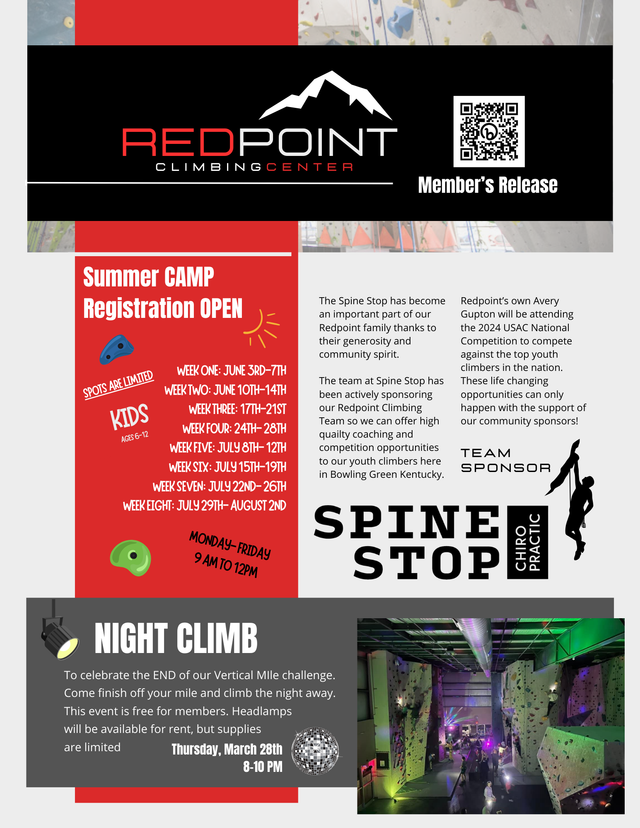The vibrant poster for Red Point Climbing Center is promoting several exciting events and opportunities for climbing enthusiasts. Dominating the poster is an announcement for the Summer Camp, which is scheduled to run throughout June and July. The camp features weekday sessions from Monday to Friday, 9 a.m. to 12 p.m., spanning eight weeks from June 3rd to August 2nd. Prospective campers can sign up using the provided registration details. 

Additionally, the poster advertises a special Night Climb event to celebrate the completion of the Vertical Mile Challenge. This free event for members is set for Thursday, March 28th, from 8 to 10 p.m., featuring a colorful night climbing experience with green and purple lights. Enthusiasts are encouraged to "finish off their mile and climb the night away," with headlamps available for rent on a limited basis. Visuals on the poster include images of climbers on an indoor rock wall equipped with multicolored handholds, cushioned landing areas, and various sponsor advertisements. A QR code is also present, allowing quick access to more information and registration options on the Red Point Climbing Center's website.